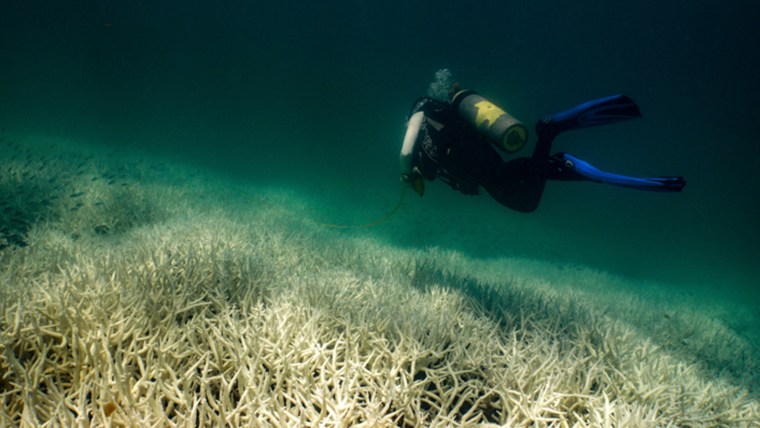The image depicts an underwater scene featuring a scuba diver near the ocean floor, which is blanketed in white coral or seagrass. The diver, dressed in a dark blue wetsuit, floats calmly just above the ocean bed. His feet are equipped with blue flippers, and he carries a large black oxygen tank adorned with a yellow design. The lighting in the scene creates a beautiful interplay of shadows and lighter areas, enhancing the serene atmosphere. Though the image predominantly captures the diver and the ocean floor, a subtle detail includes a school of small fish towards the left side of the frame. The water displays a gradient from misty green near the bottom to darker blue at the top, emphasizing the depth of the scene. Additionally, a rope connected to the diver suggests a link to the surface, possibly serving as a safety measure. The overall stillness of the scene is highlighted by the absence of larger marine life.